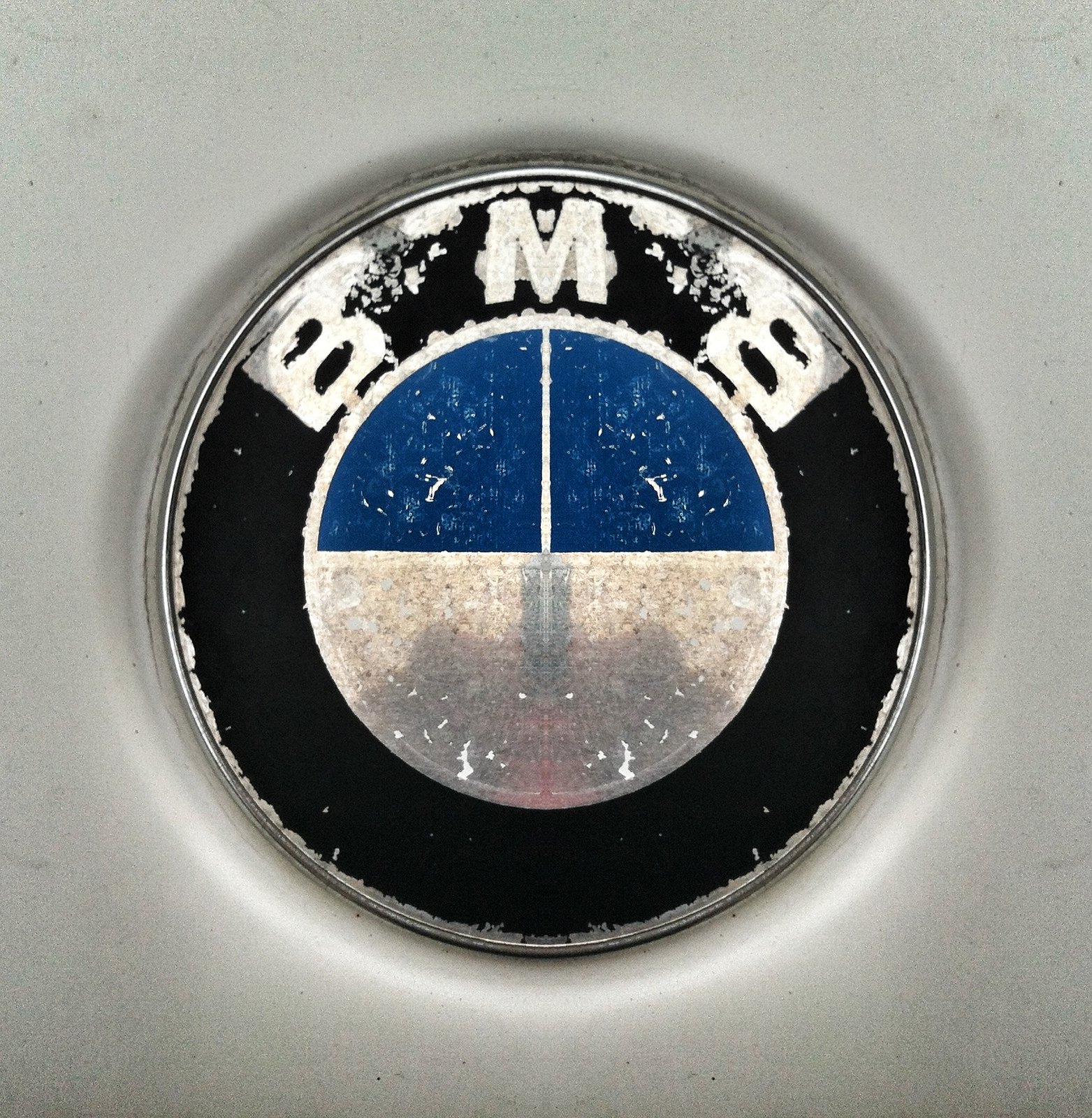The image features a worn button designed to resemble the iconic BMW car emblem. However, in this artistic rendition, the traditional "BMW" letters are replaced with "BNB," presenting a fresh and unique interpretation of the classic design. The button maintains the emblem's well-known blue and white propeller motif, but here, the blue section spans one side in a half-circle formation. The black segment, which typically houses the "BMW" lettering, now displays the letters "BNB," though they appear weathered and chipped. Set against a stark white background, the piece exudes an aura of aged elegance, reminiscent of Andy Warhol's pop art interpretations, such as his famous Campbell’s Soup Cans. The overall effect suggests a thought-provoking commentary on branding and artistic reinvention.